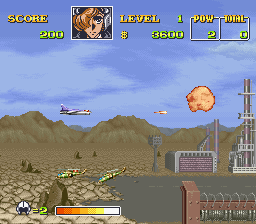This captivating screenshot from a side-scrolling video game vividly depicts an intense war scenario. The sky occupies the top half of the image, painted a vibrant blue with wispy clouds scattered throughout. Prominently featured is a silver plane at the center of the scene, in mid-flight and firing a missile. Just inches in front of the plane, the missile is about to strike, creating a striking orange explosion with red borders and a pinkish core. The backdrop includes a rugged brown mountain range and a sprawling military base. The base consists of two main grayish buildings: a tower and a structure resembling a garage, with a gray runway cutting through the terrain and a brick-colored fence.

In the game's user interface, "SCORE" is displayed in yellow lettering at the top-left, showing a score of 200 in green. Adjacent is a square featuring an image of the pilot, with one eye visible and the other obscured by hair. To the right, the text "LEVEL" appears in yellow, followed by a dollar sign with "$3600" underneath. Continuing further right, '1' is displayed above the last zero. Additionally, two boxes with white borders are visible: the first labeled "POW" with a green number ‘2’ beneath it, and the second labeled "TOTAL" showing a yellow ‘0’.

The ground below the structures presents a blend of dirt and rock formations. To the right of the military base, a slender gray road offers a stark contrast against the broken, rocky soil. Adjacent to the road, there's a fence-like structure wrapped with what appears to be barbed wire, emphasizing the war-torn setting of this intense and detailed video game scene.